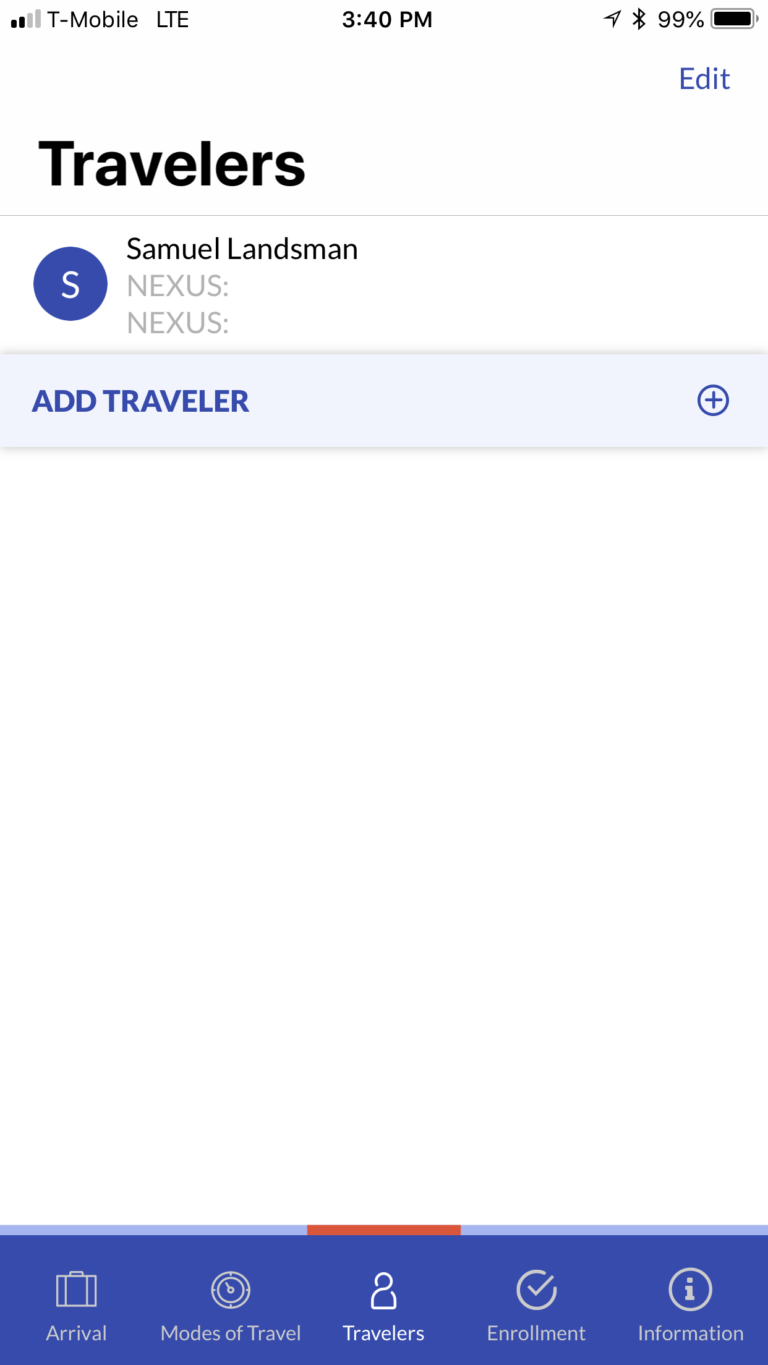"Mobile Screenshot of Travel App Interface

The screenshot portrays a travel app on a mobile phone with a clean, white background. At the bottom of the screen is a blue footer featuring five white icons with corresponding gray text labels, except for the center one which has white text. From left to right, the icons depict:

1. A suitcase or briefcase labeled 'Arrival'
2. A speedometer labeled 'Modes of Travel'
3. A person labeled 'Travelers'
4. A checkmark inside a circle labeled 'Enrollment'
5. An eye inside a circle labeled 'Information'

Above the footer, there is a light blue bar with a distinct red section in the middle. This is followed by a white background that displays the word 'Travelers' in large black text at the top. To the upper right, there is a blue 'Edit' option. A thin gray line divides this section from the one below it, which is labeled 'Information.'

On the left side of this section is a blue circle with a white 'S' in the center, adjacent to three lines of text in black and gray:
- 'Samuel Lansman' in bold black text
- 'Nexus: Nexus:' in lighter gray text beneath

Following this, there is a prominent light blue box with a soft gray shadow that contains the phrase 'ADD TRAVELER' in uppercase, bold, sans-serif text. On the right side of this box, there is a blue-outlined circle with a blue plus sign in the center.

The header at the very top of the phone screen shows the time, '3:40 PM,' centered. The top right corner displays several icons: an arrow pointing up and to the right, a Bluetooth symbol, '99%' indicating signal strength, and a nearly full battery icon filled in black."